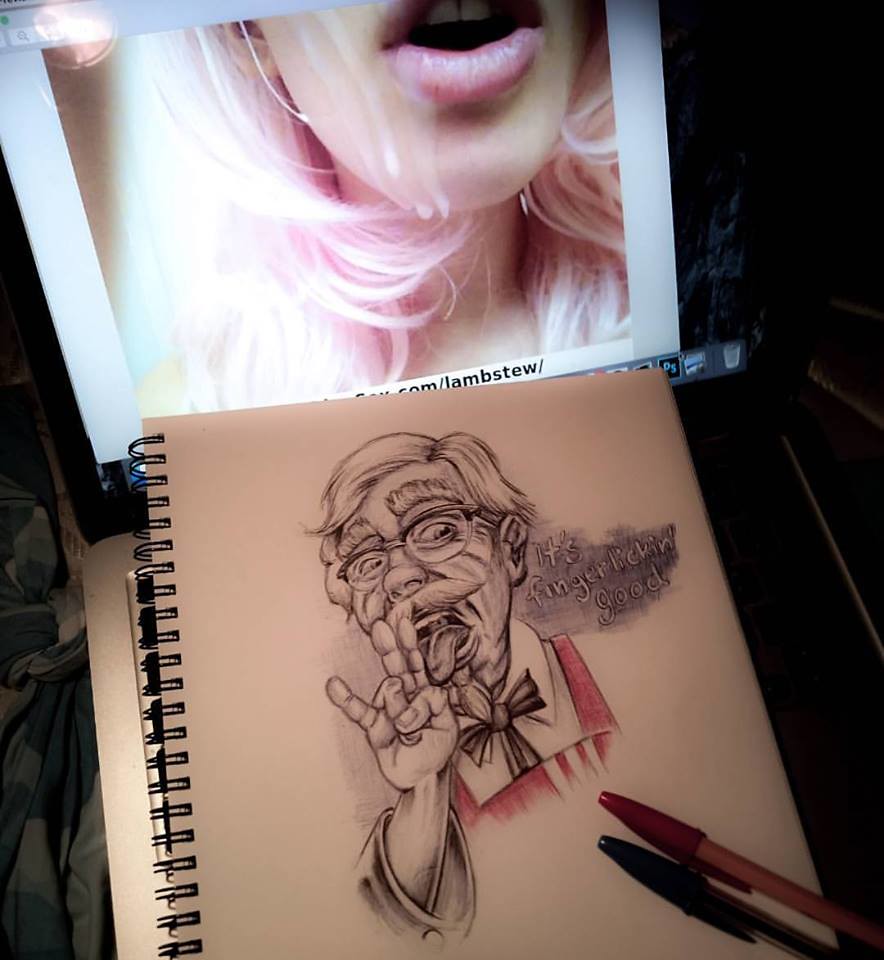This photograph, taken on a desk surface in a dark room, features an intriguing juxtaposition of images. The background is pitch black, making it difficult to discern the surrounding environment, but the edge of a desk or tabletop surface is barely visible. On the left side of the image, there's a camo-patterned green blanket piled up.

Dominating the center of the photo is a tablet propped against the wall, displaying a screenshot capturing the bottom half of a woman's face. She has very light blonde hair, almost white, with pink lipstick and white liquid dripping down her face. 

Adjacent to the tablet, there is a sketch pad with an artistic drawing of the Kentucky Fried Chicken mascot, Colonel Sanders. The illustration is created using red and black ink pens, which are visible in the bottom right corner of the sketch pad. Colonel Sanders is depicted with white hair, glasses, and bushy eyebrows, wearing his traditional apron, predominantly black with some red shading. He is making a lewd hand gesture, holding the ring finger and thumb pressed against his face while sticking his tongue out. A speech bubble next to him reads, "It's finger-lickin' good." The sketch pad's binder rings are visible along the left side, indicating it is a rip-out style book.